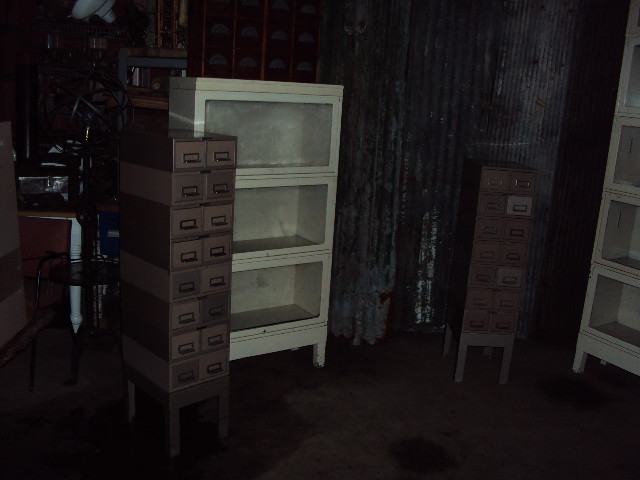The image depicts a darkened, unfinished room that looks like a basement, filled with various storage items. Prominently featured in the center is a white barrister's bookcase with glass-fronted shelves, surrounded by brown, narrow filing cabinets with multiple small drawers. There appear to be two metal card catalog cabinets, one to the left and one to the right of the bookcase, each with two columns and eight rows of small drawers. The room is partitioned by a vertical plastic curtain. The floor is a dirty concrete with wet spots. In the background, there is a clutter of additional objects, including shelves, a small table, and a red chair. The room is poorly lit, making it difficult to distinguish all the details, but a reflection of bronze and a variety of dark-colored items can be noted.